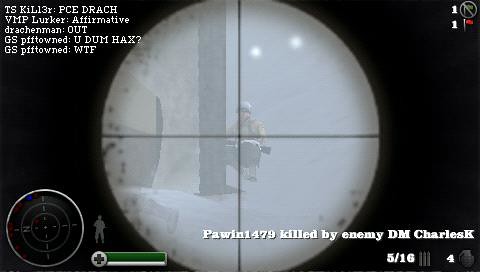This image is a detailed screenshot from a computer game. The background is predominantly black, with a large pale white circle at the center. This circle features a crisscross of vertical and horizontal lines that intersect in the middle. Positioned centrally within the circle, there is an outline of a soldier. The soldier is equipped with a white helmet, a brown jersey, and black trousers, and is nearly crouching while facing towards the crosshair, which extends to the edges of the circle.

In the upper left corner of the image, several lines of white text are visible: "TS killer TCE dredge," "if the MP Luka affirmative," "Frenchmen out," "GS if town you D max UT hex?", and "GS P PFF town WTF." 

On the bottom left corner of the screen, a map depicted as a white circuit with red and blue dots and faint lines is visible. Adjacent to it is a gray model of a person with a green health bar beneath it. In the bottom right corner, text reads, "Paween 479 killed by enemy TM chalice," which is accompanied by a "5 over 16" indicator, an upward-facing arrow, a representation of bullets, and a number "4" with accompanying grenades.

Finally, the top right corner of the image features the text "1 1" alongside a small red dot.